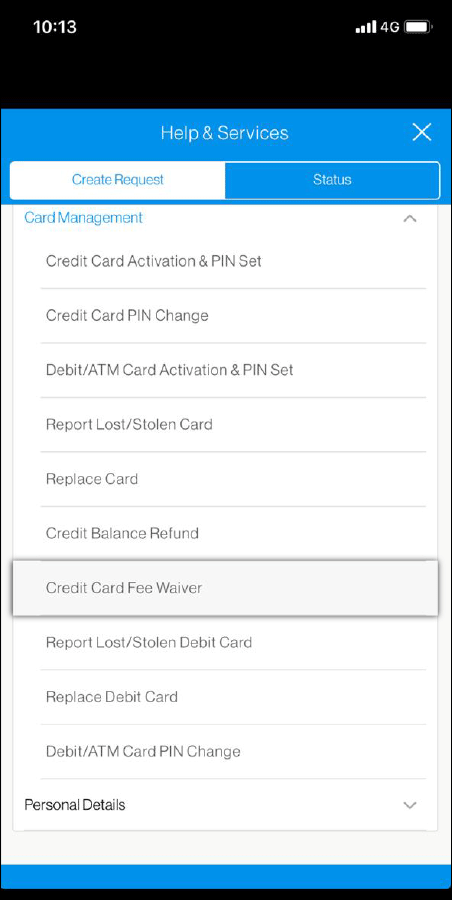The image displays a cell phone screen with a highly detailed user interface. At the top of the screen is a black border containing the time "10:13" in the upper left corner, alongside the cellular signal icon, "4G" indicator, and a battery icon aligned in the upper right corner. Directly below this is a blue border displaying the text "Help and Services" in white, with a white "X" on the far right.

The interface features two tabs beneath the blue border. The left tab is highlighted in white with blue text reading "Create Request," while the right tab has a blue background with white text that says "Status." Below the highlighted "Create Request" tab, the heading "Card Management" is presented in blue text.

Following this heading is a list of options:
1. "Credit Card Activation and PIN Set"
2. "Credit Card PIN Change"
3. "Debit/ATM Card Activation and PIN Set"
4. "Report Lost/Stolen Card"
5. "Replace Card"
6. "Credit Balance Refund"

An emphasized option, "Credit Card Fee Waiver," stands out with a slight border and a light gray background.

Continuing down the list are additional options:
7. "Report Lost/Stolen Debit Card"
8. "Replace Debit Card"
9. "Debit/ATM Card PIN Change"

At the bottom of the list, the text "Personal Details" appears in bold with a small downward-pointing arrow to its right.

The bottom of the page features a blue banner without any text, capped off with a thin black border.